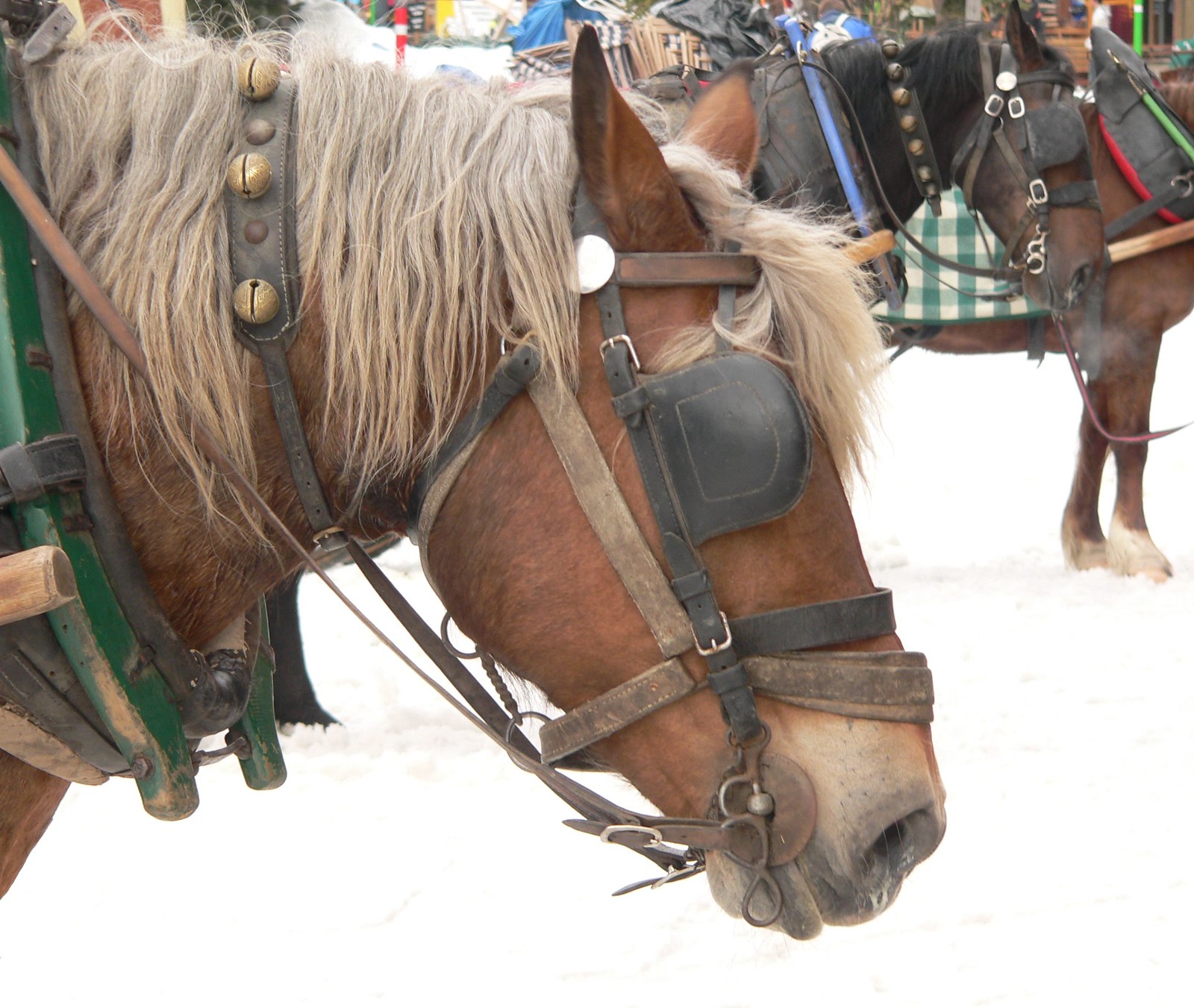In a snow-covered outdoor setting reminiscent of winter or Christmas time, this detailed image captures three horses adorned for the cold season. The foreground features a close-up of a light buckskin palomino horse, showcasing its dirty blonde mane, bridle, and distinctive blinders over its eyes. Jingle bells, fastened around its neck with a leather strap, add a festive touch. Next, a brown horse stands slightly farther back, visible from the neck down to its saddled back, which is draped with a green and cream-checked cloth. Lastly, a bay horse with white markings on its legs stands in the background, partially obscured but identifiable from its neck back. The snowy ground is trampled where the horses have moved, and faint village elements such as a green post or bench are discernible in the blurred background, contributing to the seasonal and rustic atmosphere.